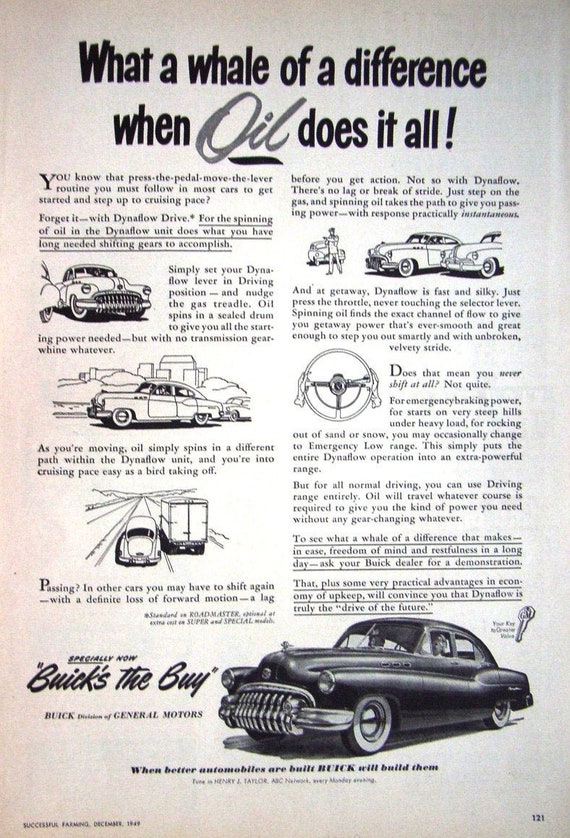The image is a vintage full-page black and white advertisement, likely from a 1950s-era newspaper or magazine, featuring the iconic Buick cars. The ad is titled "What a Whale of a Difference, When Oil Does it All," with this phrase prominently displayed at the top. The word "oil" is notably highlighted in larger, cursive, gray text, underlined in black, setting it apart from the rest of the non-cursive black text.

The body of the advertisement consists of two columns of detailed text, accompanied by illustrations of classic 1950s-style Buick cars. These vehicles are black and white, some filled in with shading for emphasis. The ad highlights various features and benefits of using oil in these cars, explaining how it enhances the vehicle's performance.

Towards the bottom of the page, a more prominently shaded, detailed illustration of a Buick is featured, suggesting it to be a highlight of the advertisement. The ad is framed with additional elements, including small text that reads, "Specially now, Buick's the buy," and a tagline, "When better automobiles are built, Buick will build them," indicating Buick's confidence in their innovation and quality. The advertisement also points out that Buick is a division of General Motors, enhancing its credibility.

There is also an image of a car key near the bottom, possibly signifying a notable innovation by Buick at the time. Overall, the ad serves as a detailed and classic representation of Buick's marketing and automotive excellence during that era.